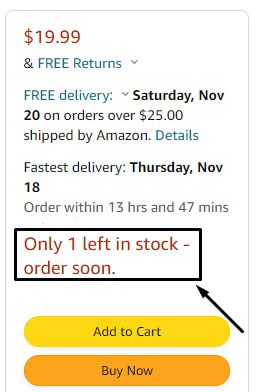In the image, there is a detailed ordering screen from a retail website, presumed to be Amazon, as it has Amazon-specific features and color schemes. At the top, it displays the price of the item as $19.99. Right below, it mentions "Free Returns" with an adjacent dropdown menu for further options. Further down, it states "Free delivery Saturday, November 20th on orders over $25 shipped by Amazon," accompanied by a clickable "Details" option. Continuing downward, it promises "Fastest delivery Thursday, November 18th" if the order is placed within the next 13 hours and 47 minutes.

The screen then features a prominent black box with the warning "Only one left in stock. Order soon." Beneath this box, there are two buttons for purchasing options: a yellow "Add to Cart" button and an orange "Buy Now" button. The layout and compact nature of the interface suggest that this is the mobile version of the Amazon ordering screen, designed to fit the dimensions of a smartphone.